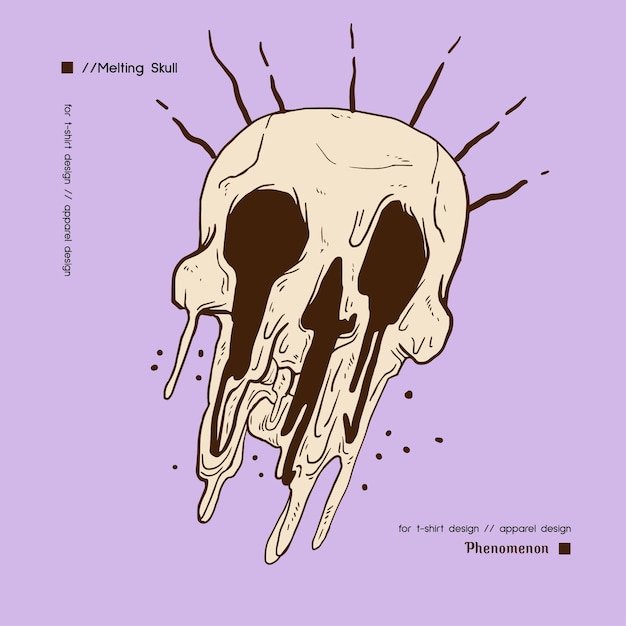This highly detailed digital illustration features a melting skull rendered in shades of cream and dark brown, set against a lavender purple background. The skull appears to be disintegrating, with the eye sockets and nose holes prominently melting into larger cavities, while the bottom portions drip into delicate droplets. Spiky, wavy lines emanate from the partially intact top of the skull, enhancing its surreal appearance. Text elements accompany the image: "melting skull" is displayed at the top left, and "for t-shirt design/apparel design phenomenon" is repeated at the bottom right, next to a black square. Additionally, a vertical inscription "for t-shirt design/apparel design" appears on the left side. The overall aesthetic mimics the effect of wax melting, emphasizing the skull’s eerie, disintegrative transformation.